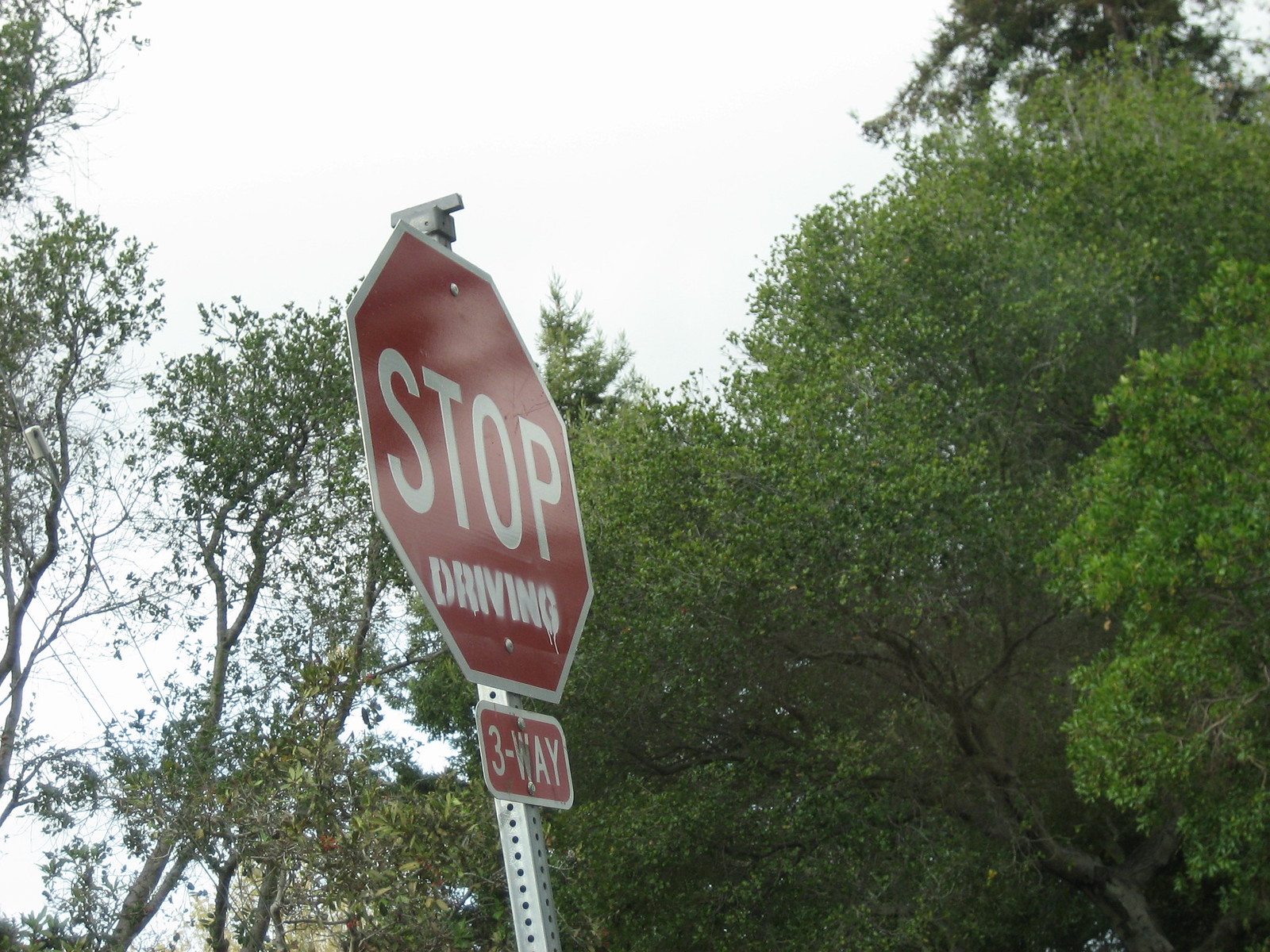This photograph captures a tilted stop sign mounted on a utility post at a three-way intersection. The sign has been visibly bumped, causing it to lean slightly to the left. Below the stop sign, another sign reads "3-WAY." In an act of vandalism, someone has spray-painted the word "DRIVING" in white stencil below the "STOP," creating a graffiti message that reads "STOP DRIVING." Paint drips are visible from the stencil. The background features lush, green old-growth trees on both the right and left sides. Utility wires and supporting guy wires can be seen on the left. The sky above is overcast, casting a light, diffused brightness across the scene.